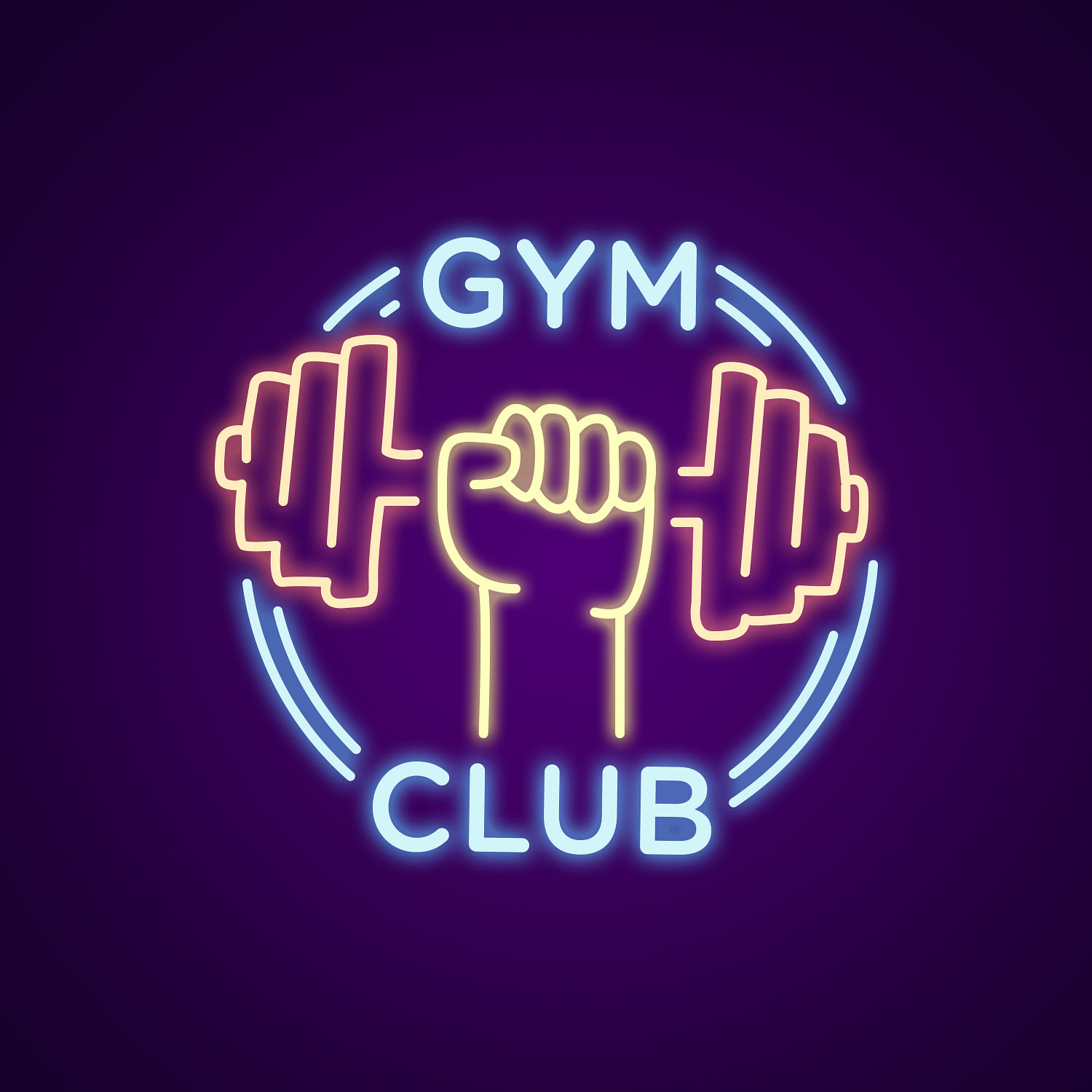The image features a square design with a dark blue background that almost fades to black at the edges, resembling a neon sign for a gym. In the center, a circular logo reads "Gym" at the top and "Club" at the bottom, both in glowing blue neon script. The circular pattern connecting the text is also blue and is interrupted by a detailed depiction of a yellow hand, shown with all five fingers tightly grasping an orange dumbbell, which has three weights on each side. The hand and dumbbell have a neon glow, with the hand outlined in the same color as the dumbbell. The logo's smooth, digitally animated design gives it a gentle neon glow, creating a visually striking gym club emblem.